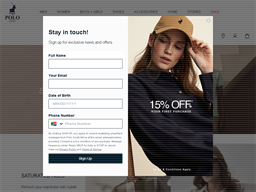This image captures the Polo online store's interface, albeit in a compact and partially obscured format. The photograph is rectangular, slightly longer horizontally than it is tall, with a greyed-out background due to a dominant pop-up in the center. In the top left corner, the Polo icon, likely in blue, is faintly visible, accompanied by some subtitles, though they are not the image's focal point.

The central portion of the screen hosts an image that's largely hidden by the forefront pop-up. Similarly, there's another image at the bottom of the screen with a caption that seems to start with "Saturday," though the full text is obscured.

The centerpiece of the image is a pop-up, formatted as two portrait-oriented photos placed side-by-side to create a square-like display. The left segment of the pop-up features a white background with blue text prompting visitors to "Stay in touch." Below, there are input fields for "Full Name," "Your Email," "Date of Birth," and "Phone Number," each accompanied by a white text box and a blue "Sign Up" button.

The right segment showcases an advertisement featuring a slender woman with long brown hair, wearing a brown Polo cap embellished with a blue logo. She is dressed in a long-sleeved blue shirt that appears to be a raincoat. A white watermark overlaying her image promotes "15% off," serving as an enticing call-to-action for potential customers.